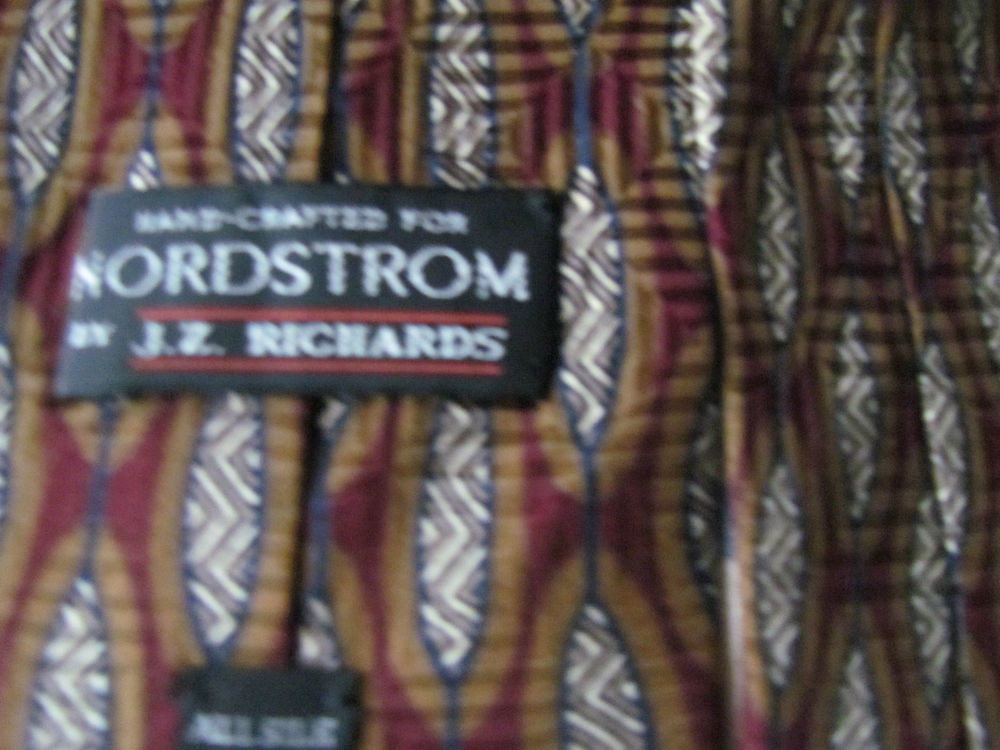This is an indoor color photograph of a close-up on a piece of clothing, focusing on a label. The image is somewhat blurry but well-lit, capturing the textured details of the fabric. In the upper left section of the image, there is a prominent rectangular tag with a black background and bold white capital letters, reading "handcrafted for Nordstrom by J.Z. Richards." Two thin horizontal red lines frame the name "J.Z. Richards" on this label. The fabric itself features a dynamic pattern comprising multicolored elements: gray and white zigzags, tan lines interwoven with maroon, and additional vertical stripes blending shades of brown, purple, and blue. At the bottom of the image, there's another smaller, nearly unreadable tag that could indicate the size. The intricate and varied pattern suggests this might be the inside of a high-quality garment such as a shirt or sweater.